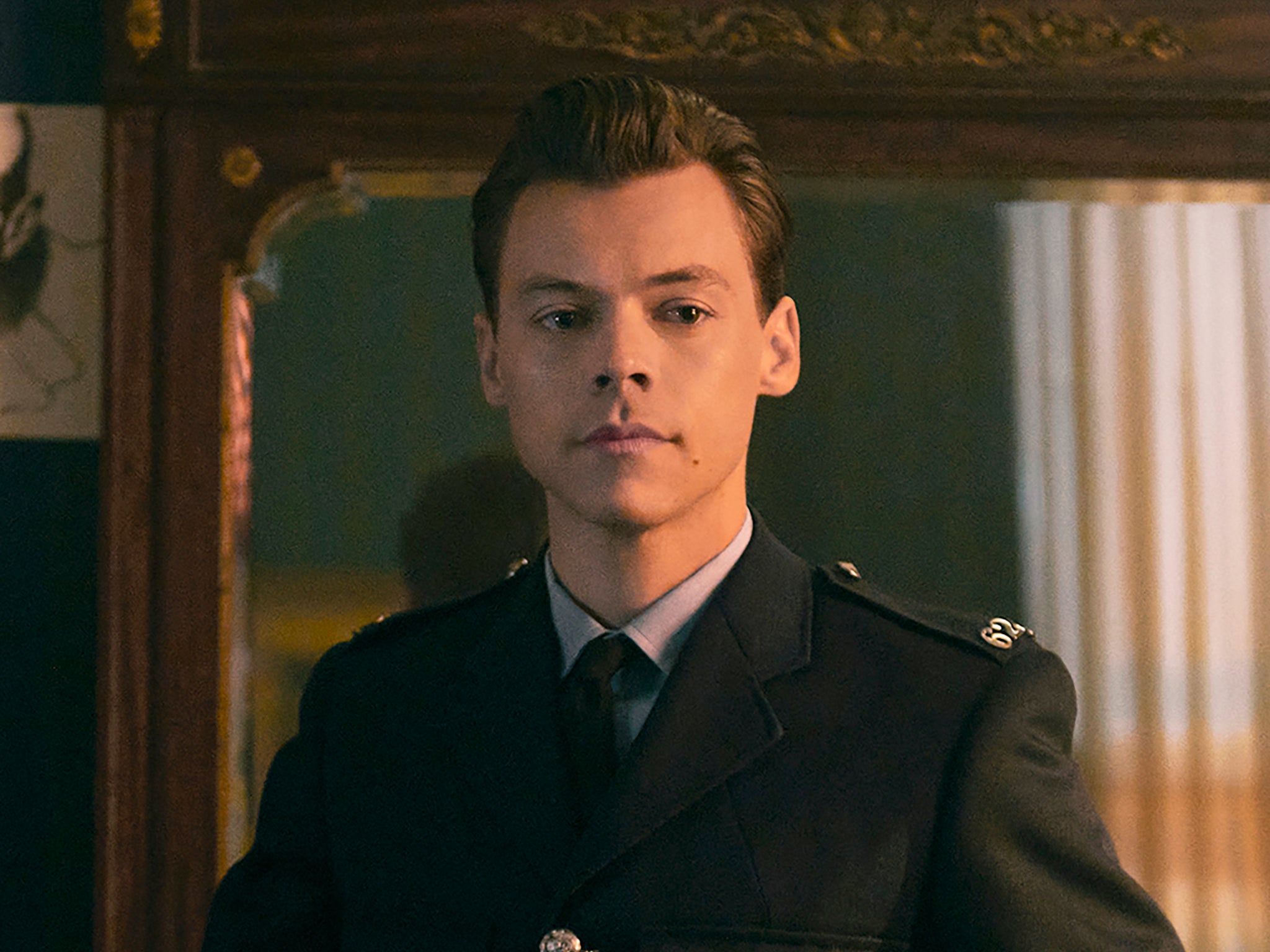This detailed photograph features Harry Styles, the main lead singer of One Direction, portraying a character on what appears to be a movie or music video set. He is dressed in a formal military-style coat, complete with a white shirt and tie. His hair is cut short and styled back, and he has a neutral, relaxed expression as he gazes slightly off to the side, away from the camera. The setting appears to be a bedroom, with a dark wood vanity and attached mirror behind him, reflecting a subdued, blurry background. A warm, orange-hued light, reminiscent of a sunset, illuminates one side of his face while casting shadows on the other, adding depth to the scene and accentuating the tranquil environment.